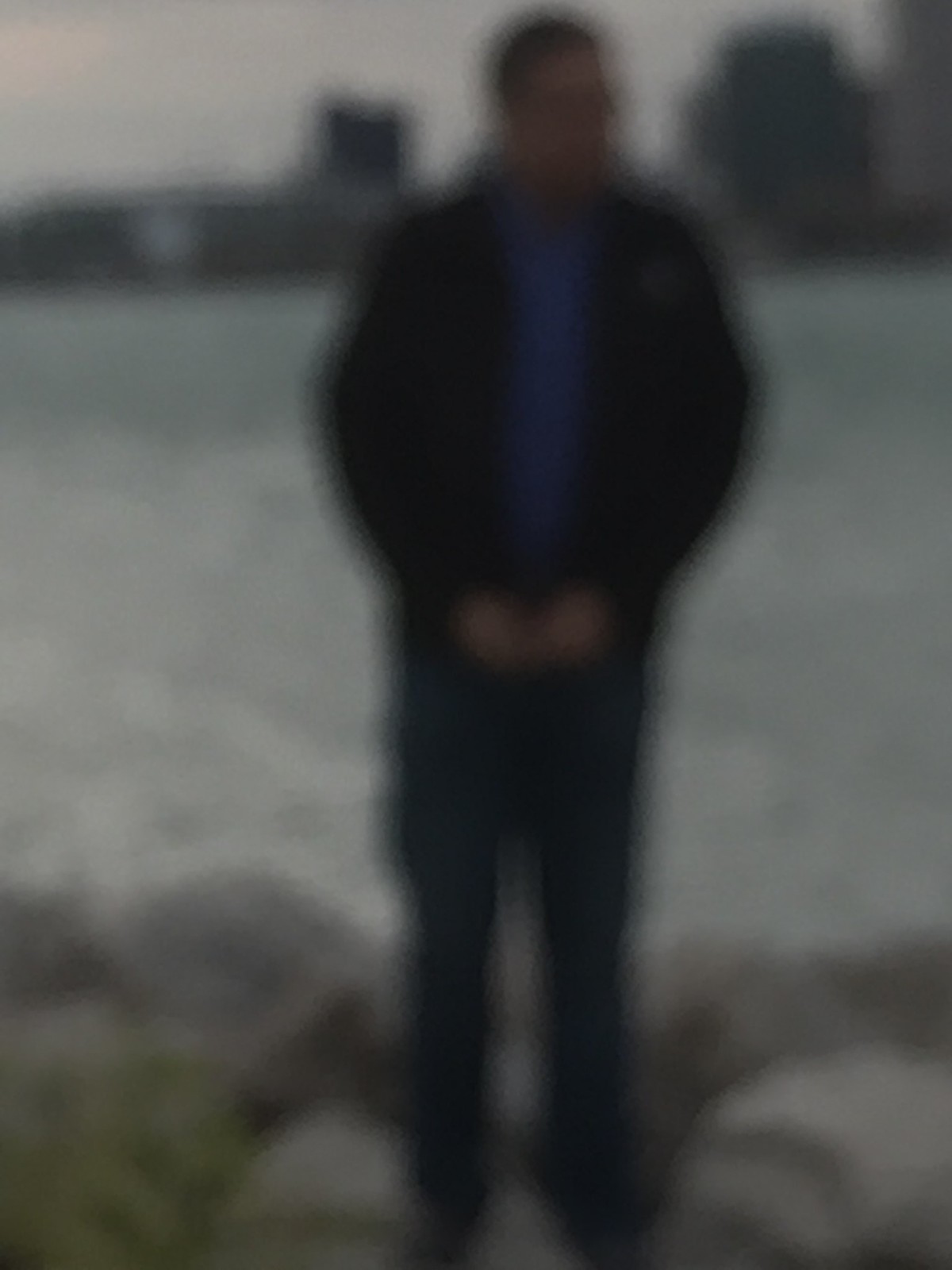A slightly blurry photograph depicts a man standing outside on a rocky shoreline, with a backdrop that includes several buildings across a body of water, possibly a river. The man appears to be Caucasian and may be in his early 40s, distinguished by his low-cut dark brown hair and eyeglasses. He is dressed in a black jacket layered over a blue button-down shirt, paired with blue jeans and dark shoes. The scene suggests he is standing near the water’s edge, perhaps on a riverbank, with the urban landscape faintly visible in the distance behind him.